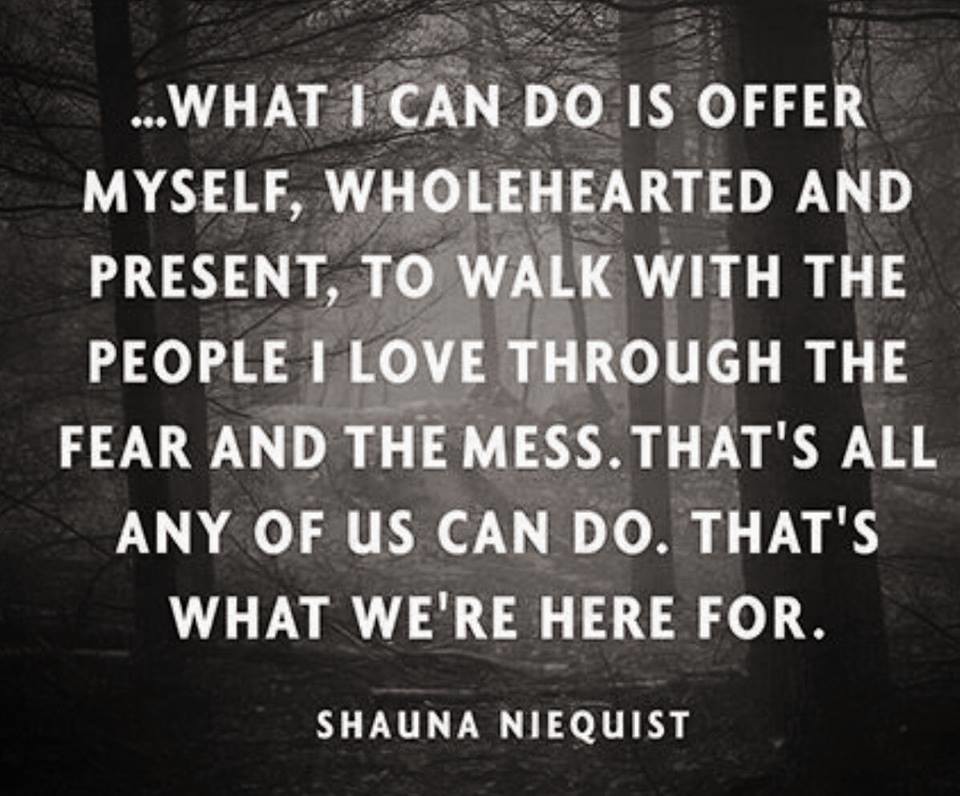The image depicts a motivational quote written in white, all-capital letters. The text, attributed to Shauna Niequist, reads: "WHAT I CAN DO IS OFFER MYSELF WHOLEHEARTED AND PRESENT TO WALK WITH THE PEOPLE I LOVE THROUGH THE FEAR AND THE MESS. THAT'S ALL ANY OF US CAN DO. THAT'S WHAT WE'RE HERE FOR." The background is a hazy, foggy forest scene in black and white, featuring bare, dead-looking trees, possibly in winter. The forest ground is visible with some scattered branches, creating a contemplative and somber atmosphere that complements the quote's message of support and resilience.